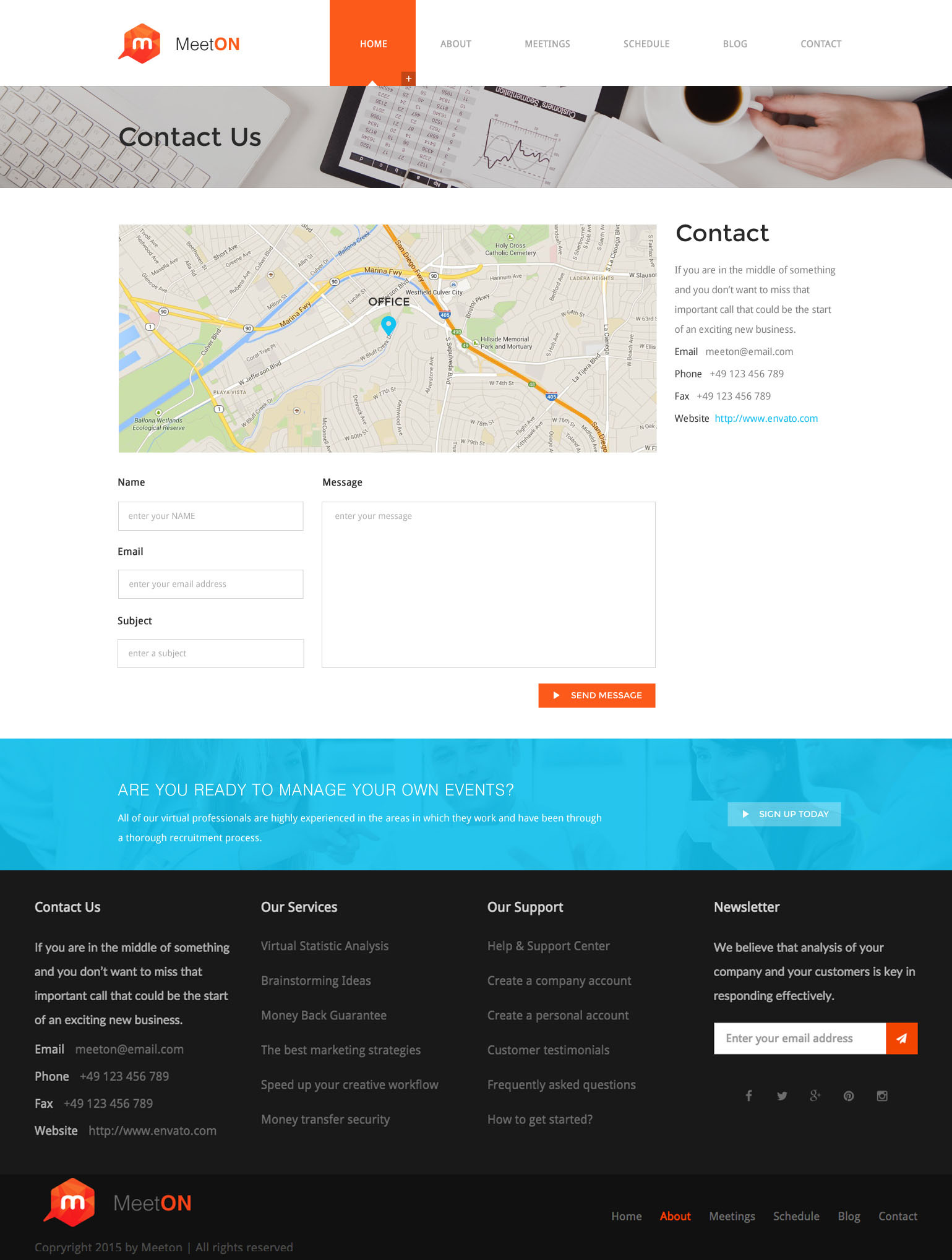This screenshot depicts the homepage of a website for a service designed to help set up events electronically. The logo, prominently featured, consists of a purple cube, turned at an angle, with a white "M" on it, followed by the text "MEET ON." The word "MEET" is in black with mixed upper and lowercase letters, while "ON" is rendered in orange and all capital letters.

The top navigation bar includes links labeled "MEET HOME," "ABOUT," "SETTINGS," "SCHEDULE," "BLOG," and "CONTACT." The "CONTACT" link is highlighted in orange, indicating the current page. Beneath the navigation bar, a banner with "CONTACT US" is displayed prominently.

The main content area showcases a map pinpointing the office location with a detailed "CONTACT" section below it. There is a paragraph outlining contact information, along with fields for visitors to input their name, email address, subject of their message, and the message itself. An orange "SEND MESSAGE" button is provided for submitting inquiries.

Below this contact form, there is a blue, rectangular banner with the headline "ARE YOU READY TO MANAGE YOUR OWN EVENTS?" followed by a brief description. Beneath this banner, in a black section, the webpage is segmented into four parts: "CONTACT US," "OUR SERVICES," "OUR SUPPORT," and "NEWSLETTER."